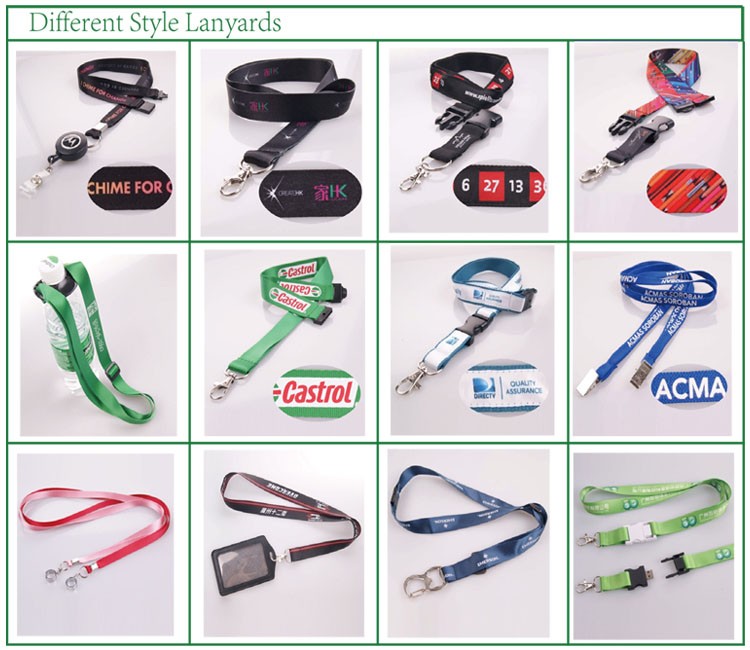The image is a large square grid composed of 12 equally-sized smaller panels, arranged four across and three down, each depicting a different style of lanyard against a gray background. The title "Different Style Lanyards" is prominently displayed in green text at the top. The lanyards in the top row include three black varieties with the fourth being a red and blue lanyard. The middle row features predominantly green lanyards, including one with the brand name "Castrol," followed by two blue lanyards; one labeled "ACMA" in white letters, and another with a "Quality Assurance DIRECTV" sign. The bottom row showcases a red lanyard in the first position, succeeded by a black lanyard equipped with a photo ID holder, then a blue lanyard, and finally a green lanyard on the far right. Each individual lanyard is distinctly highlighted within its own small square panel, contributing to the cohesive design of the grid.